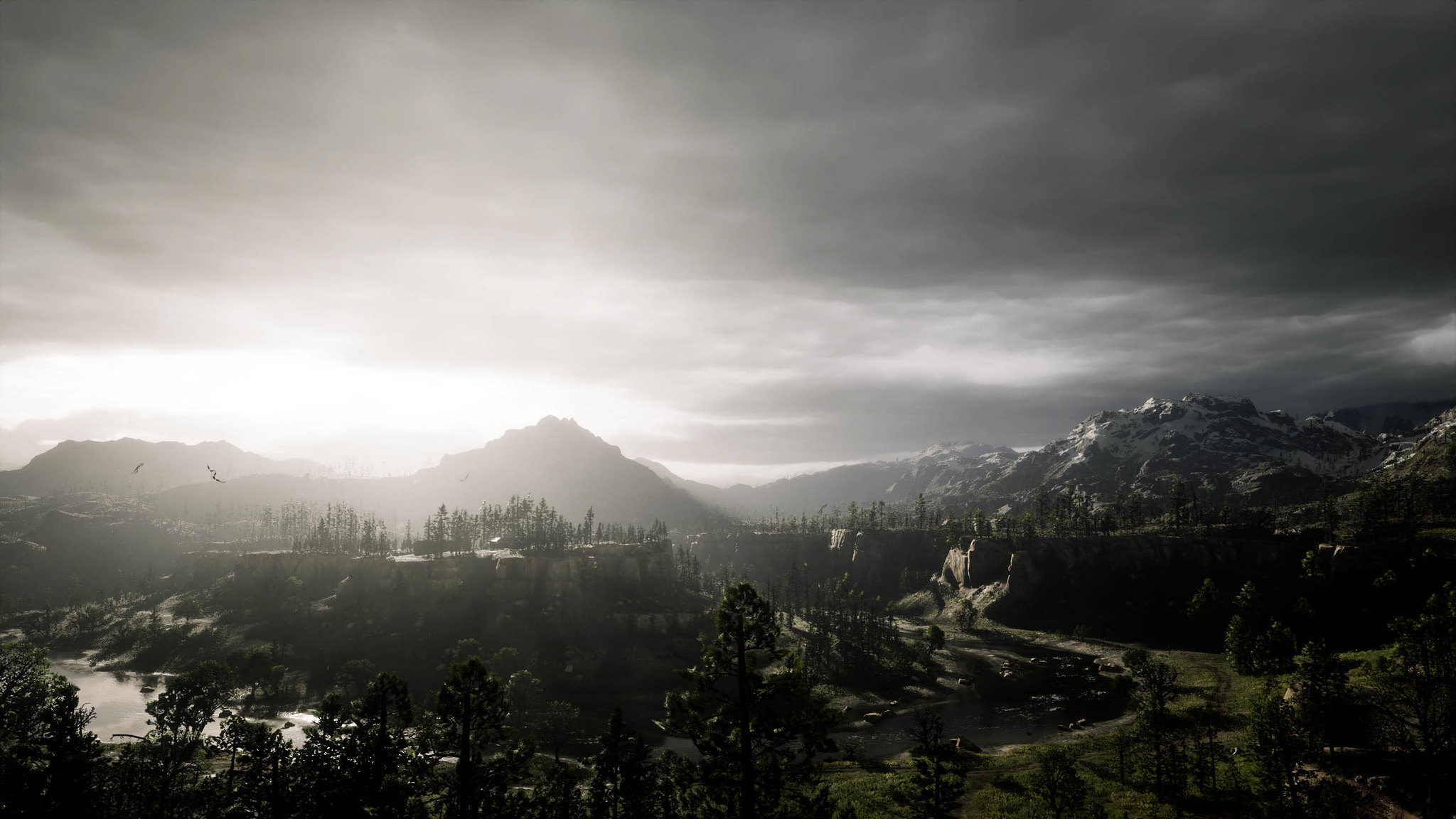The image presents a breathtaking, potentially computer-generated or heavily photoshopped landscape with a predominantly black, white, and gray color palette. The scene captures a vast, mountainous, forested area. The sky, heavily clouded, transitions from dark gray clouds on the right to lighter clouds on the left, suggesting dynamic lighting and shadows that might hint at a CGI origin. Sunlight appears to be piercing through some of the clouds, creating a dramatic and bloomy light effect in the background. Below the sky, the left side of the image features a water body, possibly a lake, surrounded by dense, dark green trees. To the right, a more open and green landscape stretches out. Dominating the backdrop are mountains which to the right are snow-capped and shown in more detail, whereas on the left, the mountains appear as a dark, rocky silhouette. The overall scene exudes an otherworldly beauty, intensified by the monochromatic color scheme and suggestive of an enhanced, surreal quality.